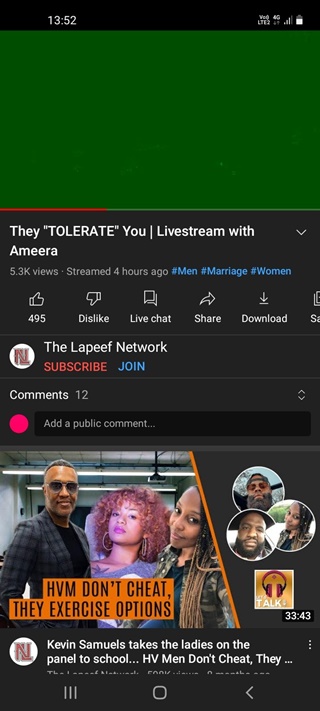The livestream thumbnail, captured on a mobile device with a full battery and 4G connectivity, shows a snapshot from a recent broadcast by Amira. The stream, titled "Men, Marriage, Women," attracted 533 views and was aired 4 hours ago. It has garnered 405 dislikes and 12 comments so far. The engagement options displayed include live chat, sharing, downloading, upvoting, and downvoting, represented by respective icons.

The image features a man with short hair, dark skin, glasses, and a black coat alongside a woman with curly hair and large loop earrings. On the right side, another woman is depicted with braided hair. The background displays lights and dials at the top, suggesting a studio environment. The overlay text includes "HVM" and phrases like "don't cheat" and "they exercise," indicating topics discussed during the stream. There are also references to a gaming channel that engages women in a metaphorical "paddle to school," and mentions of "corona" and "HV men."

The layout includes visual cues like a green square, public comment sections, and several icons such as a right circle and a downward arrow. The environment appears busy and detailed, aligning with the thematic elements of relationships and societal norms discussed in the livestream.